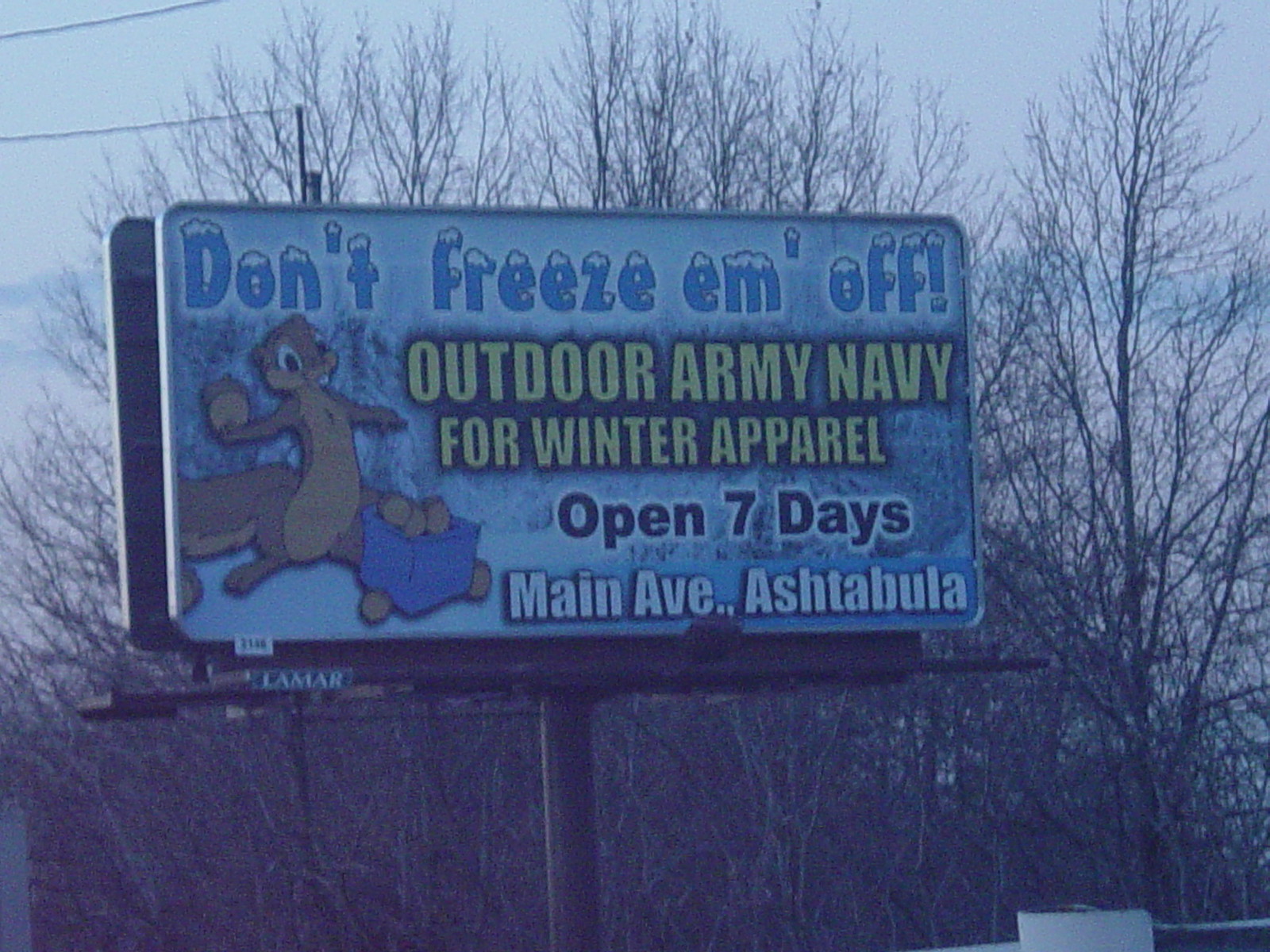"Captured on a clear daytime, this photograph showcases a roadside sign promoting winter apparel at Outdoor Army Navy. The sign humorously alerts passersby with the phrase, 'Don't freeze them off,' and provides details about being open seven days a week at Main Avenue, Ashtabula. On the left side of the sign, an illustrated chipmunk is depicted holding an acorn in its right hand, seemingly ready to toss it into a small blue box filled with acorns at its feet. The background reveals a forest of bare trees, highlighting the seasonal change as fall transitions into winter."